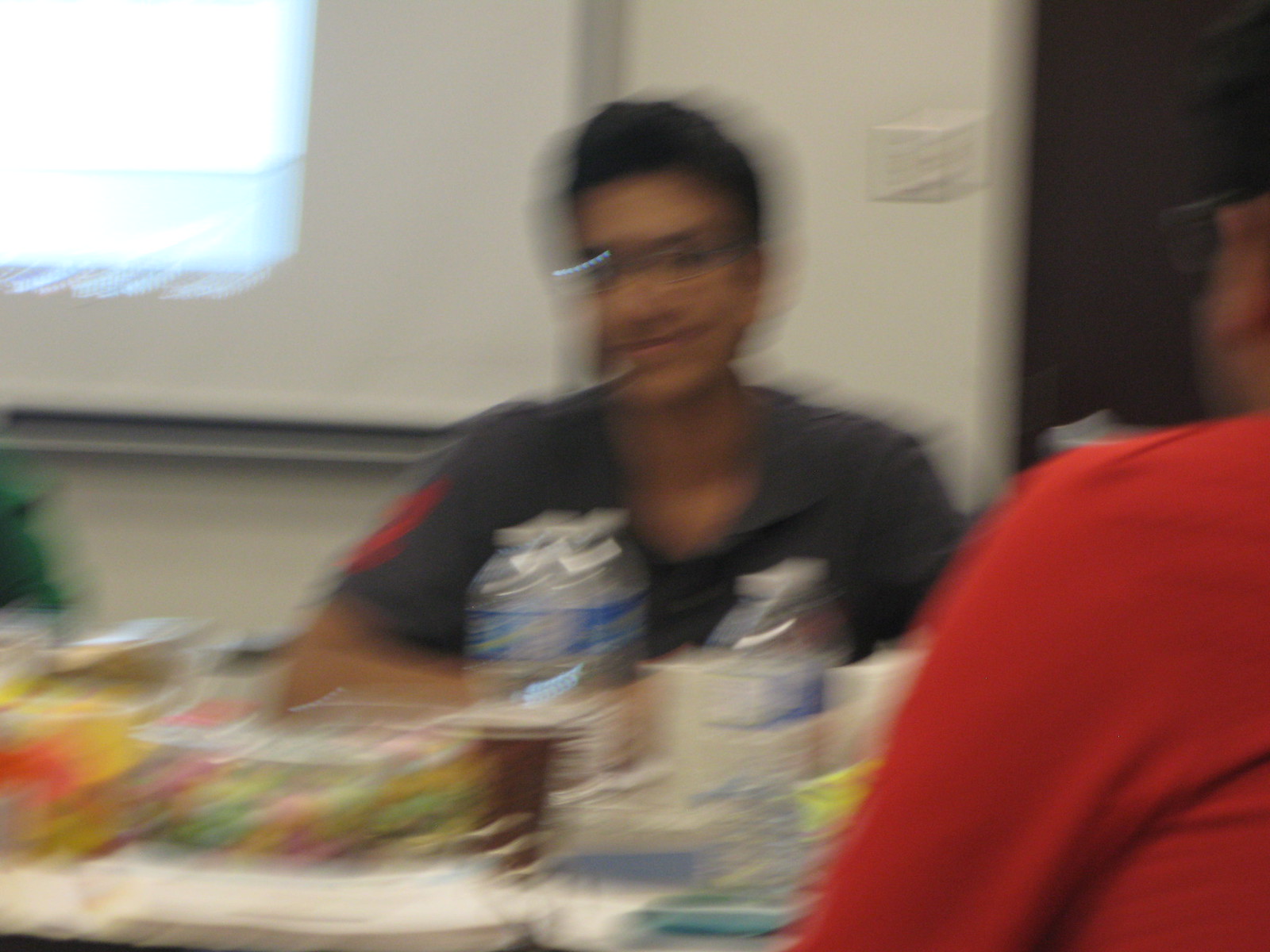A photograph, taken in landscape format during the daytime with natural light, captures an indoor setting. Despite its low resolution and motion blur, the image reveals two individuals engaged in interaction at a table laden with food and drinks. The person in the foreground, shown from the back on the bottom right side of the image, wears a red long-sleeved shirt, glasses, and has dark hair with darker skin. He faces away from the camera, focusing on the individual across the table. The second person, situated centrally and looking directly into the camera, sports a gray short-sleeved shirt with a red logo on the right shoulder, suggesting a uniform. This individual also wears glasses, has short dark hair, and exhibits a warm smile. The table, white in color, is cluttered with various items, including water bottles, plastic food boxes with vibrant contents, and possibly a coffee cup. In the background, a light switch can be seen on the wall, and a bright window with overblown highlights is visible in the top left corner. Given the setting and details, it appears to be a casual or break room environment.